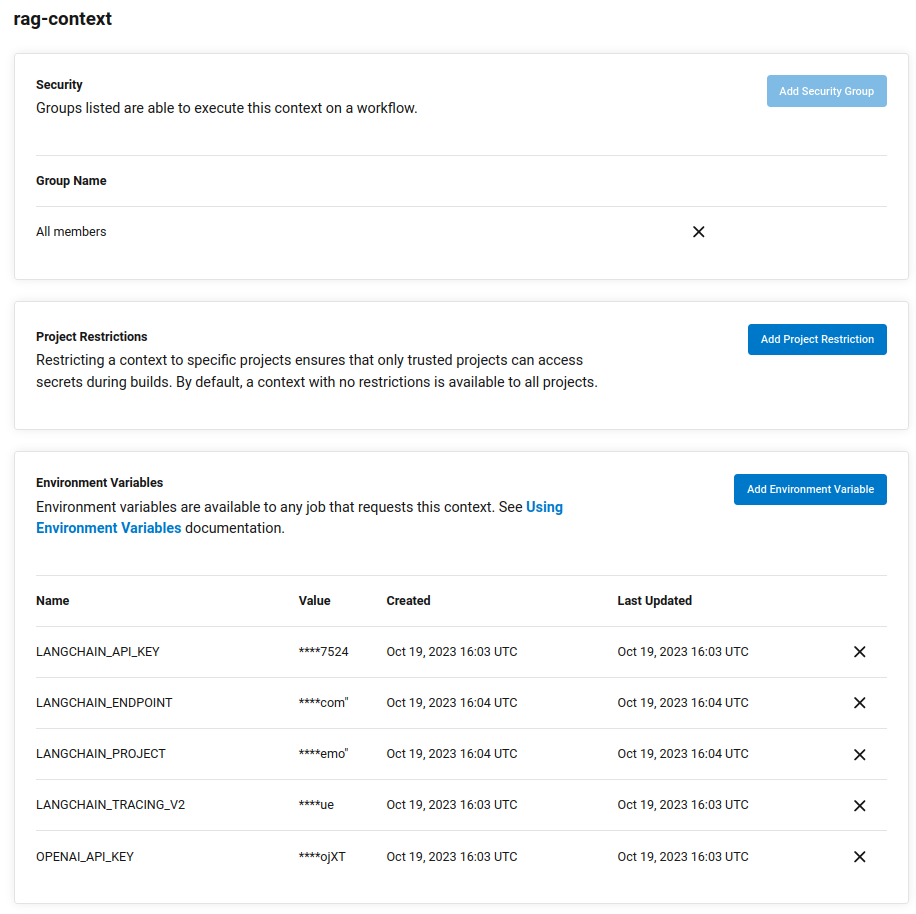Sure, here's a detailed and cleaned-up caption for the image based on the provided voice input:

---

The image depicts a detailed configuration interface for managing security contexts within a workflow. The "RAG context security groups" section allows administrators to list and manage specific security groups enabled to execute this context. There is an option to add a new security group, wherein you'd specify the group name and its members. For instance, the group name could be 'All Members', denoted by the identifier 'X'.

In the "Project Restrictions" section, administrators can restrict the context to certain projects. This measure ensures that only trusted projects have access to sensitive secrets during build processes. If no restrictions are set, the context will be available to all projects by default. To add a project restriction, click the 'Add Project Restriction' button.

The "Environment Variables" section provides an overview of environment variables that any job requesting this context can access. For detailed guidance on using these variables, refer to the "Using Environmental Variables Documentation". Administrators can add new environment variables, specifying their name, value, creation date, and last updated timestamp. An example entry is an environment variable named 'Lang Chain API Key' with the value '7524', created and last updated on October 19th, 2023, at 16:03 UTC.

---

This caption provides a clear, structured explanation of the different sections and functionalities displayed in the image.